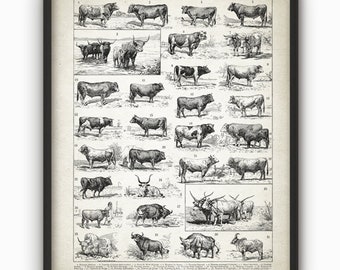The image features a small, highly detailed diagram hanging on a white wall, centrally framed in a thin black frame with inner shadows and vertical pinstripes. The artwork showcases dozens of finely sketched cows, steers, and possibly buffalo, all depicted in various shades of gray on a cream-colored background. The sketches, arranged in rows and pairs, highlight different breeds and characteristics, including solid-colored and spotted dairy cows, and distinct horned varieties. Each animal is meticulously numbered and labeled, though the small size of the image renders the specific text and numbers difficult to read.